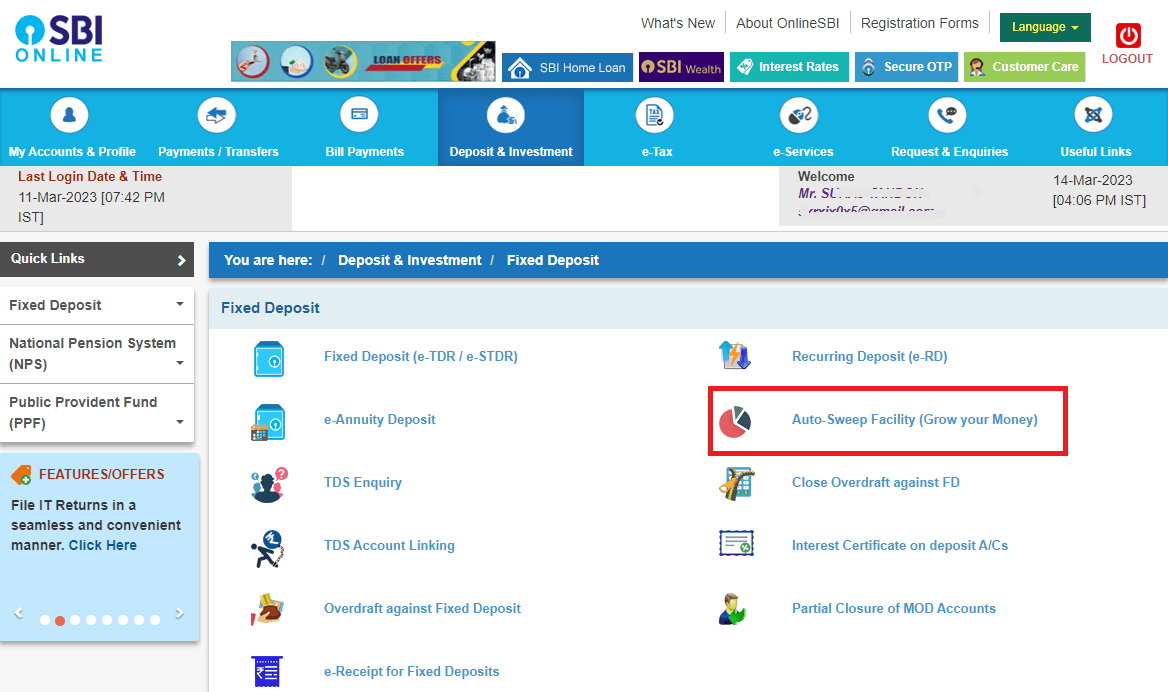The image showcases a retro-styled online banking interface for SBI, featuring a navigation bar at the top with a light blue background. Key sections in the navigation bar include "My Accounts and Profile," "Payments/Transfers," "Bill Payments," and "Deposits." A prominent advertisement for loan offers appears near the top of the screen. On the left-hand side, there are quick links to various services like Fixed Deposit and National Pension System.

The main focus of the screen is the "Payments/Transfers" section, specifically under the "Fixed Deposit" category. Options available here include Fixed Deposit, E-Annuity Deposit, TDS Inquiry, Recurring Deposit, Close Overdraft, and Interest Certificate. A box is highlighted around the "Auto Sweep Facility" option, which includes a note to "Grow Your Money" in parentheses. The overall design invokes a nostalgic, old-fashioned feel but is modern in functionality.